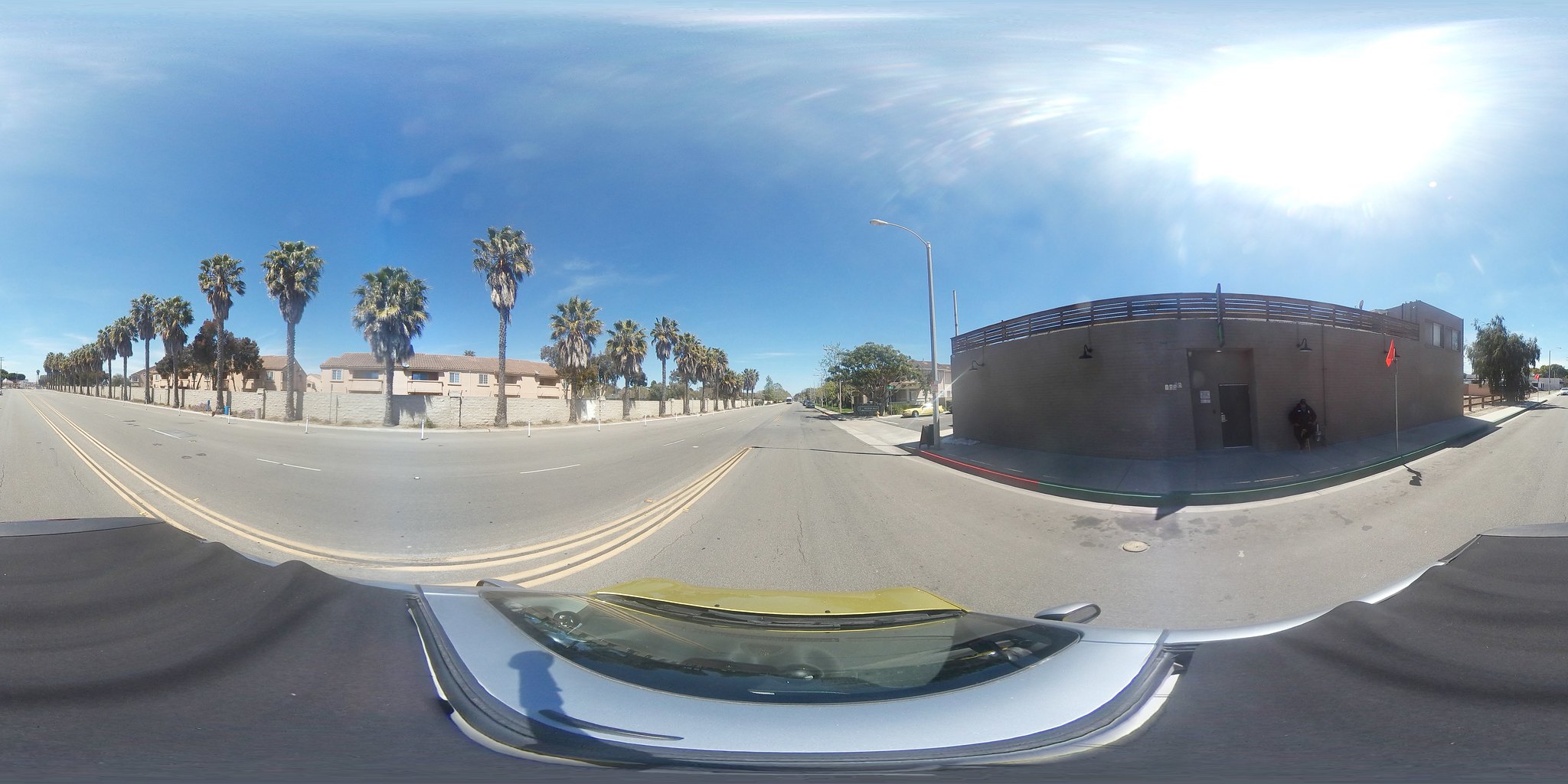On a relatively clear day with scattered clouds and ample sunlight, this image captures a panoramic view featuring various buildings and natural elements. On the left side of the image, there's a peach-colored apartment complex with a darker roof, complemented by several palm trees enclosed within a structure resembling a brick fence. To the right, a dark gray building stands, against which an individual is seen reclining. The image is taken with a fisheye lens, offering a wide, nearly 180-degree perspective. Centrally positioned in the scene is a notable gray object with a glass-like top, encircled by a substance that appears to have a gray, foam-like texture. The scene unfolds on a road, with evident shadows cast by the sun, highlighting features like an orange-flagged pole on the right.